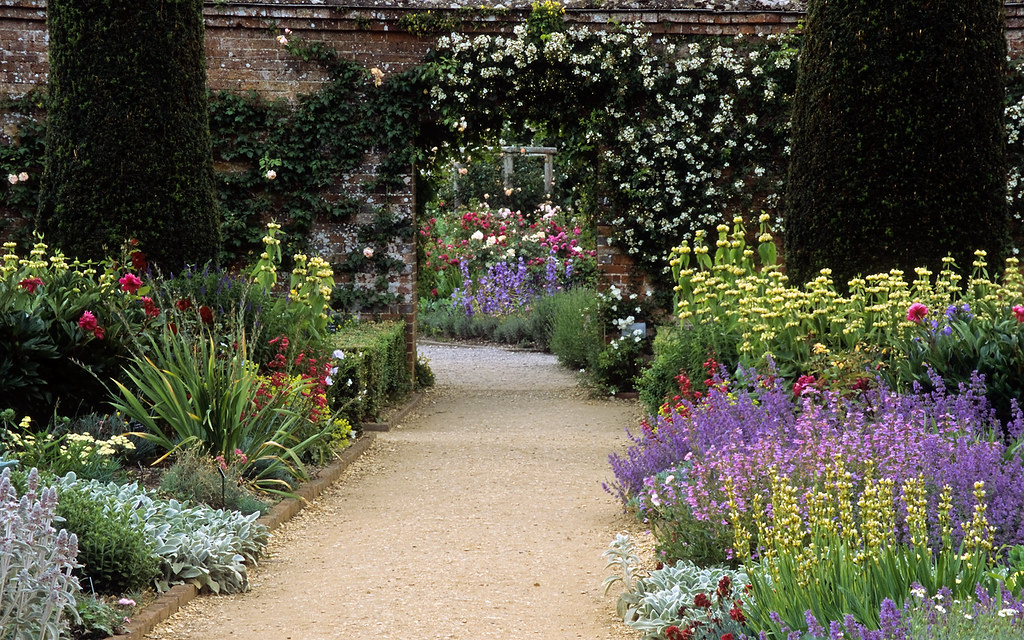The image depicts a beautifully landscaped flower garden centered around a tan, crushed stone pathway that meanders through a vibrant collection of flora. On the left side of the path, various bushes and greenery are interspersed with white flowers and grasses, creating a lush and inviting atmosphere. Further back, a tall bush adorned with pinkish flowers adds a touch of color. The right side of the path is a striking kaleidoscope of vibrant blooms, starting with purple lavender followed by bright yellow flowers, pink flowers, and clusters of small white flowers near the front. Dominating the scene towards the background is an elegant archway enveloped by lush green vines and white flowers, which frame an opening in a red or off-red brick wall. To either side of the archway, approximately six feet from the walkway, stand two tall evergreen trees or large bushes, also entwined with green vines. The overall effect is one of meticulous beauty, with a harmonious blend of colors and textures, creating a serene and enchanting garden vista.